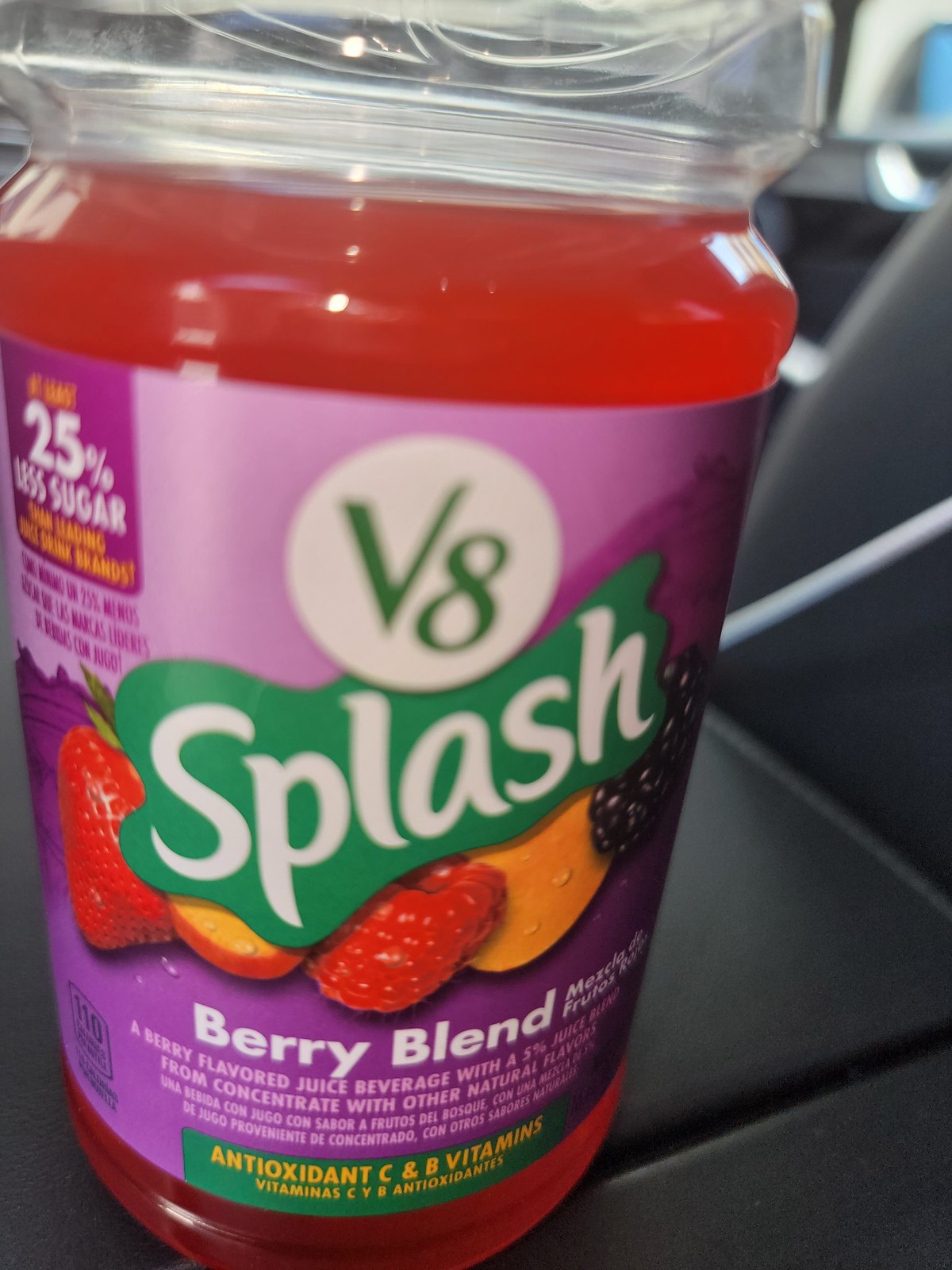This image shows a close-up of a clear plastic bottle of V8 Splash Berry Blend set against a dark surface, likely a car seat. The bottle is filled with a peachy-red liquid. The label, predominantly in light and medium purple tones, prominently displays the V8 logo inside a white circle at the center, with "SPLASH" in white text against a green splash-like background. The label highlights several types of fruits, including strawberries on the left side, a peach slice at the bottom left, a raspberry towards the bottom, an orange slice at the bottom right, and a grape on the right. 

The label indicates that this beverage contains 25% less sugar, is flavored with 5% juice from concentrate plus other natural flavors, and provides antioxidant C and B vitamins. Nutritional information such as "110 calories" can also be seen. The text includes both English and Spanish descriptions, noting the drink as "Berry Blend" and "Mezcla de Frutas." The overall presentation of the product emphasizes its fruity flavors, nutritional benefits, and reduced sugar content.